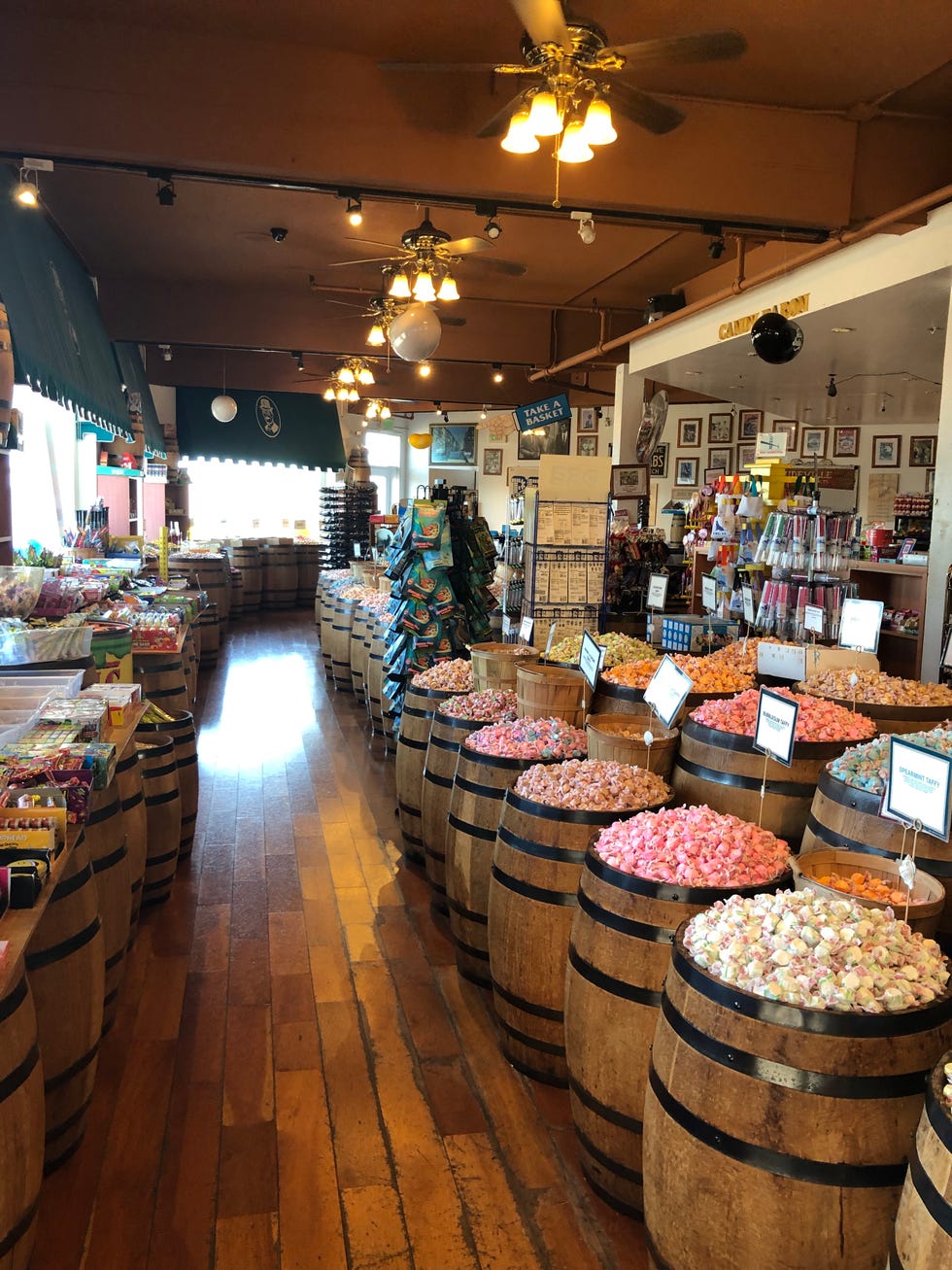This image captures the cozy interior of a country-style convenience store filled with a myriad of goodies. Dominating the view are several wooden barrels, each turned upright with their tops removed, revealing an assortment of colorful products inside—possibly various types of popcorn or candy. The items range in color from white, pink, beige, and brown in the front barrels to orange, darker tan, bluish-green, and pink in the back. Every barrel has tags for identification, though the details on them are unclear.

The store features wooden floors that complement the rustic charm conveyed by the barrels. Towards the back, additional items for sale are neatly arranged on shelves and rolling racks, including candies and potentially chips. The walls are adorned with numerous pictures, possibly showcasing products or decorative elements, adding to the store's inviting atmosphere.

Illuminating the space are ceiling fans equipped with four lamp lights each, casting a warm glow. Further to the left, studio lights line a prominent horizontal black bar under the ceiling. Black covers shield the windows from the harsh midday sun, reducing heat and glare inside the store. A clearly legible cyan sign encourages customers to "take a basket," enhancing the welcoming, shopper-friendly vibe of this charming retail space.